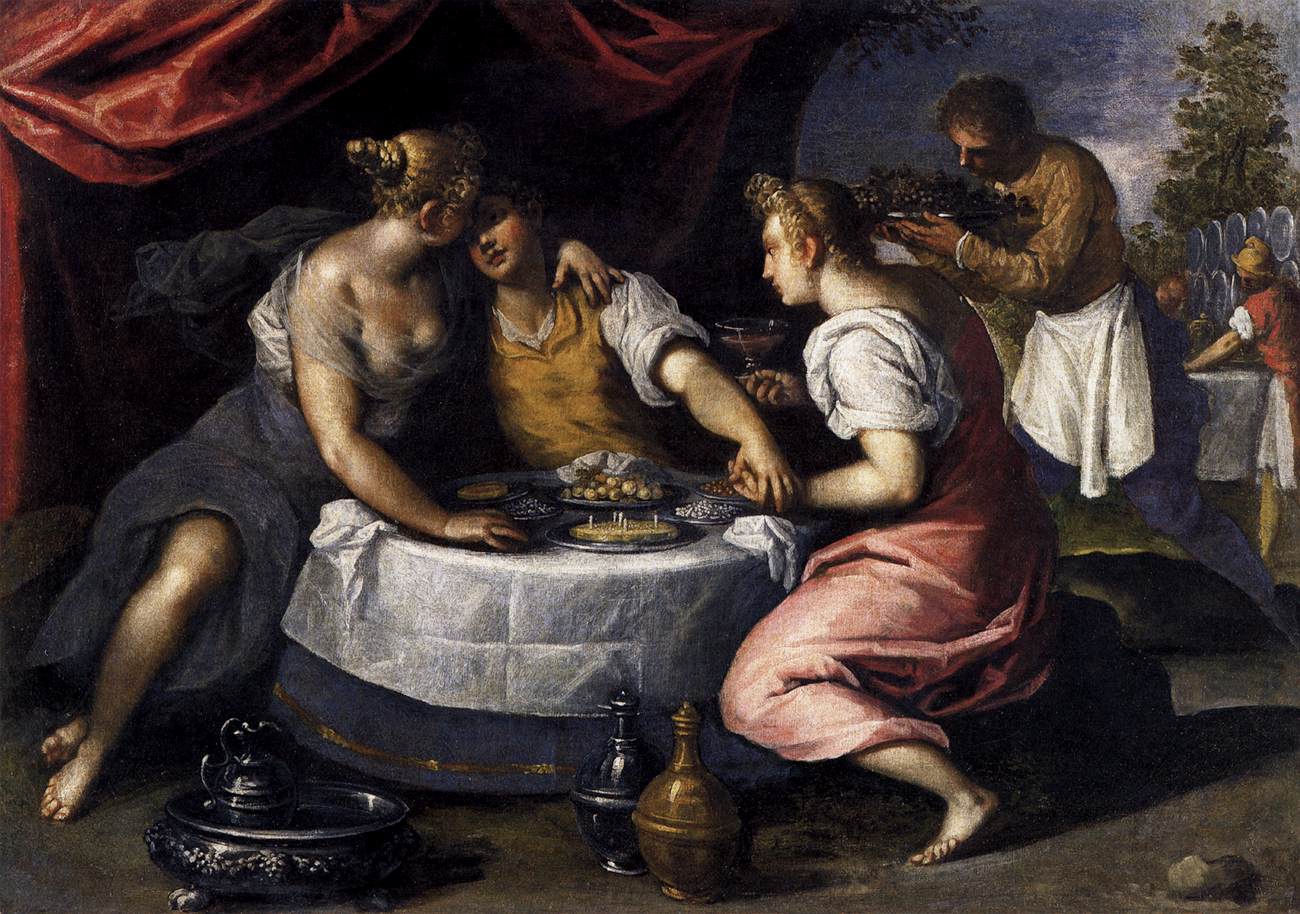This dramatic, horizontal, Renaissance-style painting captures an intimate scene set in an old-world restaurant. The composition is dominated by dark tones with sharp contrasts of white light, enhancing the emotional depth. In the foreground, under the glow of an evocative, dark background, a round table draped in a white tablecloth is decked with food and tableware. The central figures include two women and a man engaged in a tender moment.

On the man's left is a woman in a dark blue skirt and a semi-transparent ribbon top, barefoot, with her hair neatly put up. She cradles the man's head on her shoulder and kisses his forehead, while her other arm rests on the table. Opposite her, a second barefoot woman, dressed in a red skirt and a white shirt, stoops down beside the table, intimately holding the man's hand. The man, clad in a tan vest over a blue and white striped shirt, his sleeves rolled up to his elbows, appears connected to both women.

The background reveals more details: a male server in a white apron stands poised with a tray, ready to approach, while another woman, likely a server too, lingers nearby. Additional figures and tables populate the scene, contributing to the bustling atmosphere. Enhancing the setting's authenticity are the red curtains in the top-left corner, alongside various objects placed near the table on the floor—a brass bottle, a black bottle, and a black basin with a pitcher, adding texture and intrigue. The overall ambiance suggests a rich narrative, captured through meticulous detail and emotive contrasts.